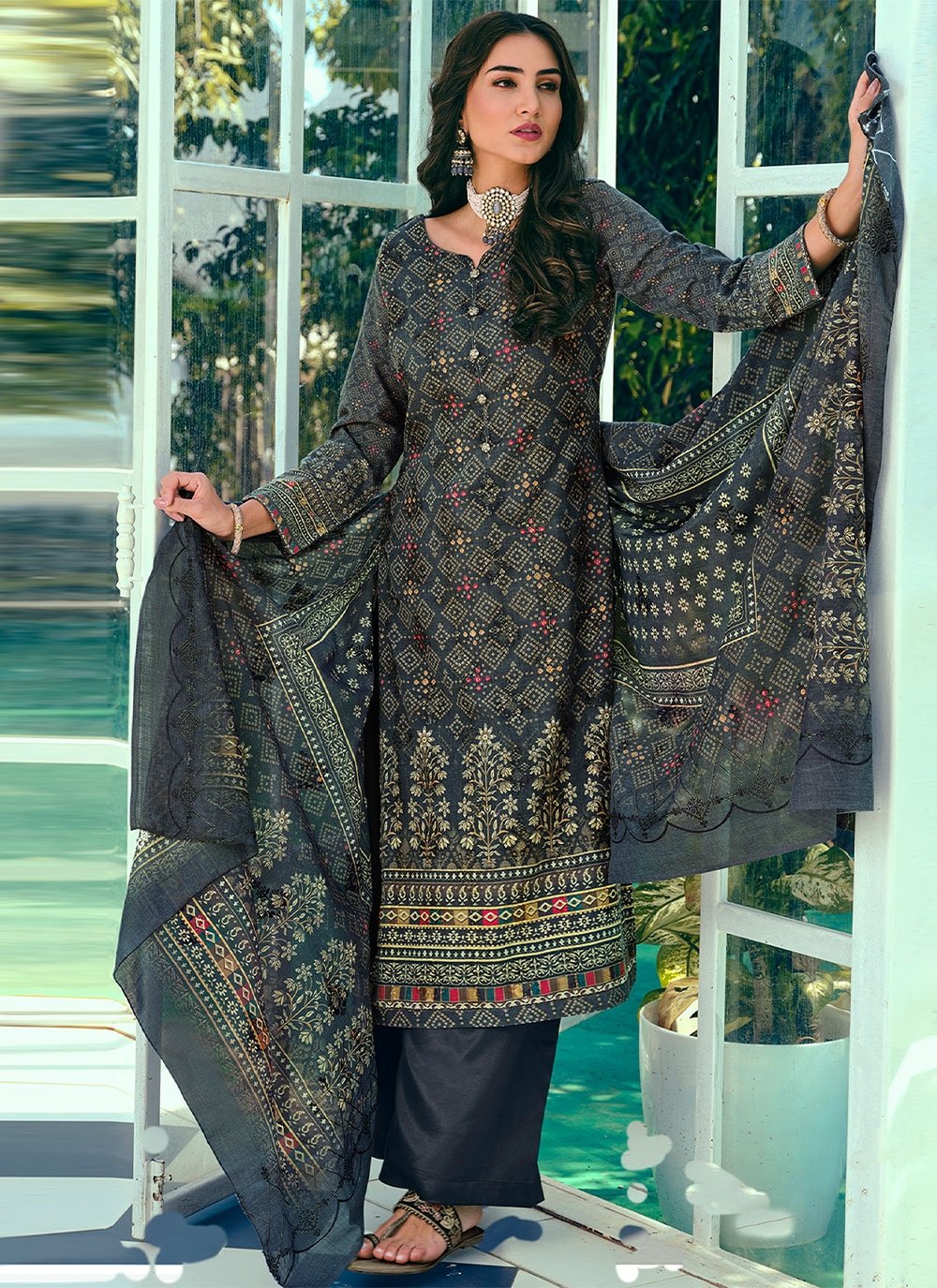A woman, likely of Indian descent, is featured at the center of this vertical photograph. She is standing in front of a framed glass door, leaning her left arm on the door frame. She wears an elaborate black saree adorned with diamond and floral patterns in brown, gold, red, orange, green, and yellow. Her attire includes a pair of black patterned slippers. She accessorizes with a layered pearl necklace and matching earrings. Her dark brown hair cascades down her back. There is no text visible in this vivid and colorful modeling photo.